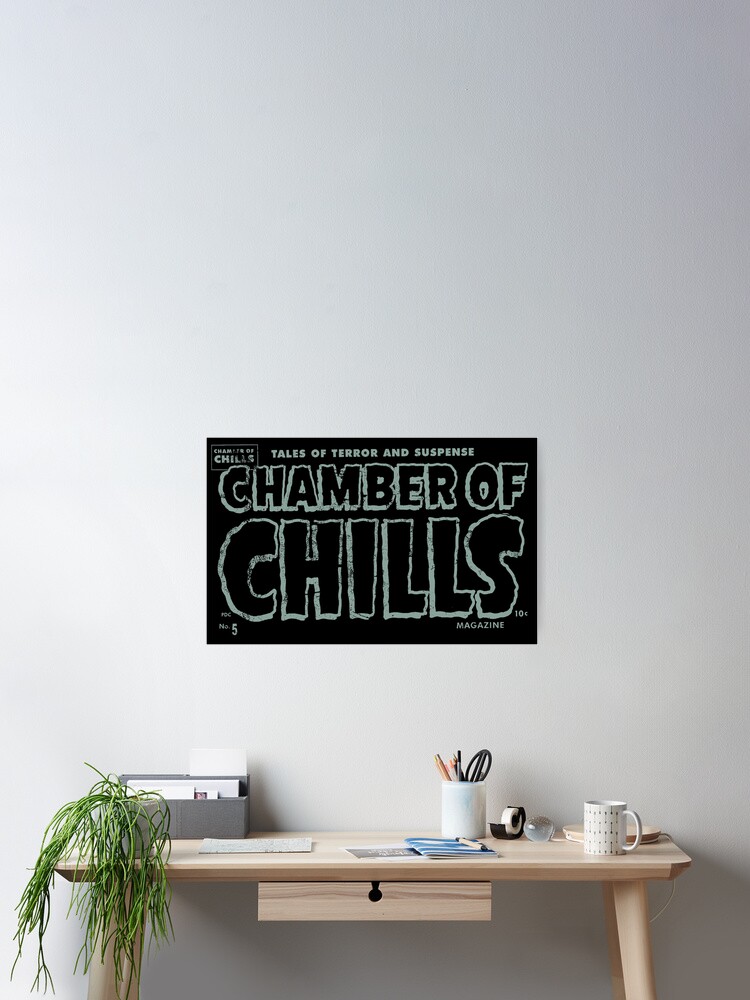This image portrays a small, light wooden desk with four slightly angled legs and a functional drawer beneath. The desk is neatly arranged with a series of items: moving from right to left, there's a white dust lamp with an L-shaped design that hangs towards the center, a coffee cup, a black tape holder, and a small glass ball. Positioned next is a white jar holding scissors and pencils. In the middle of the desk, there's a brochure or notebook accompanied by what seems to be a picture. To the far left, a plant—likely a spider plant—with green branches draping over the edge of the desk. Above the desk on a lilac-colored wall, a black and gray horizontal sign reads, "Tales of Terror and Suspense" at the top and "Chamber of Chills" in larger letters below. The writing on the sign is in a slightly grayish, bluish block style. This home office setting contrasts sharply, with the feminine, minimalist desk and its decor clashing with the bold, eerie aesthetics of the poster above it.